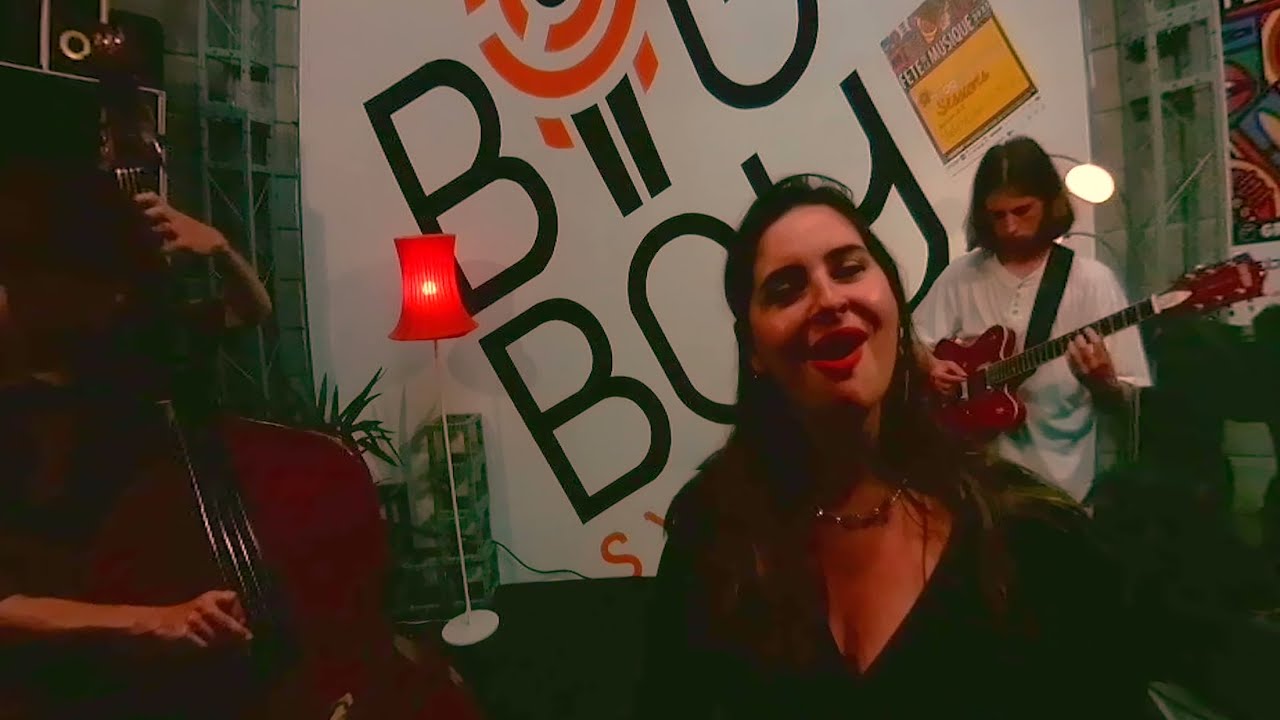This indoor photograph showcases a musical performance by a band on stage. Central to the image is a female lead singer, identifiable by her long dark brown hair, red lipstick, and black shirt. Her mouth is open, suggesting she is singing. To her right, there is a male guitarist with chin-length hair, playing an electric guitar. To her left, a cellist is visible with part of their instrument. The backdrop features a large white sign with partially obscured text, including "Big Boy" and "Fête de Musique," hinting at a French connection. Additional details include a red lamp on the left side near the cellist and visible speakers behind the performers, enhancing the atmosphere of an intimate live music setting.